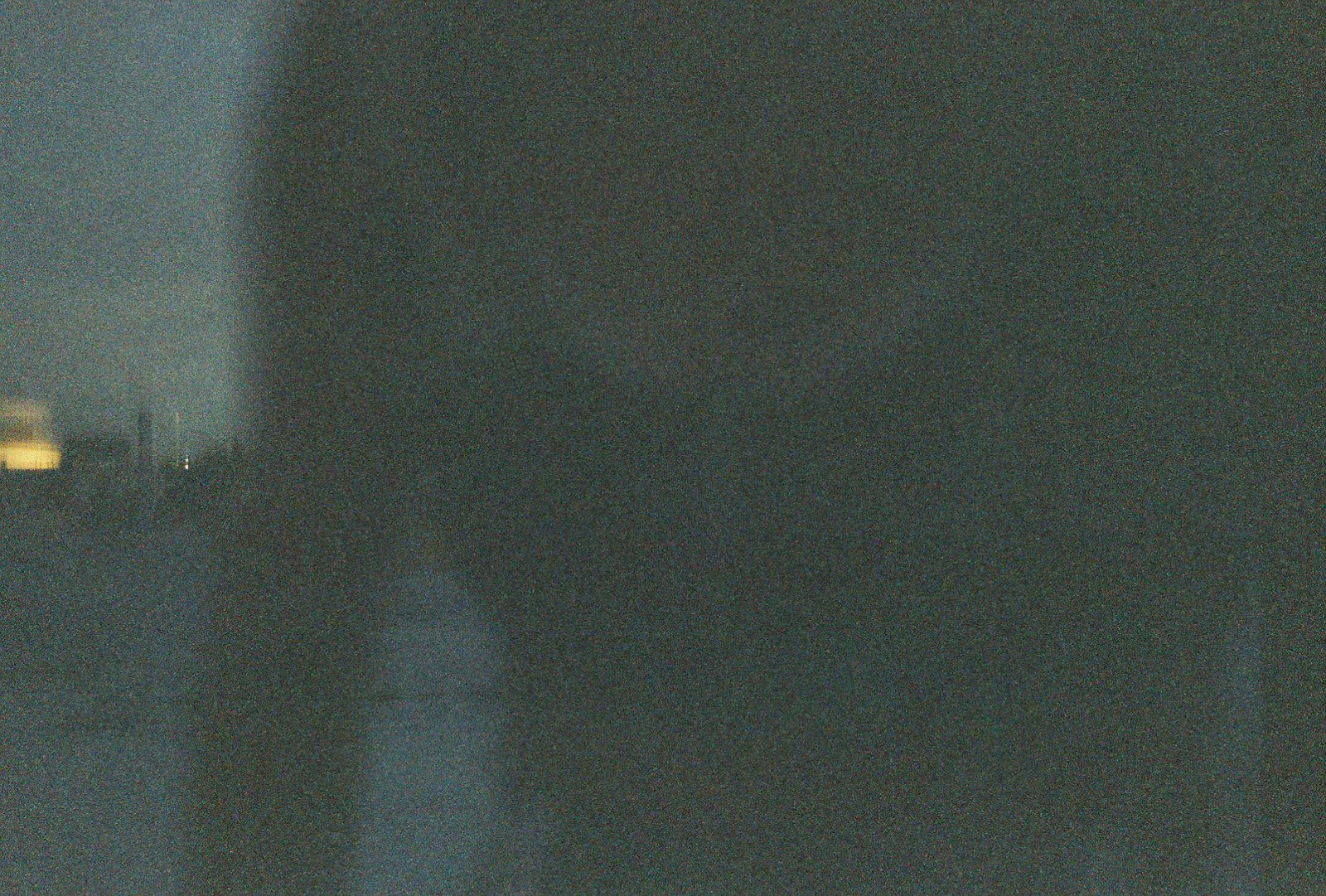The image appears to be taken from inside a building, looking out through a window that has a greenish tint, possibly due to low resolution or a filter. Reflected on the window is the chest and arms of a large human figure, though the upper part of the body is not visible. The reflection dominates the central part of the image. In the background, to the left, one can see a faint blue and white sky, suggesting a cloudy day. Below the sky, there is a discernible yellow light, which could be from a nearby building. Additionally, there is a small tower-like structure visible in the distance, and a gray street running along the bottom part of the image. Everything appears slightly faded, making it challenging to discern finer details in the scene.